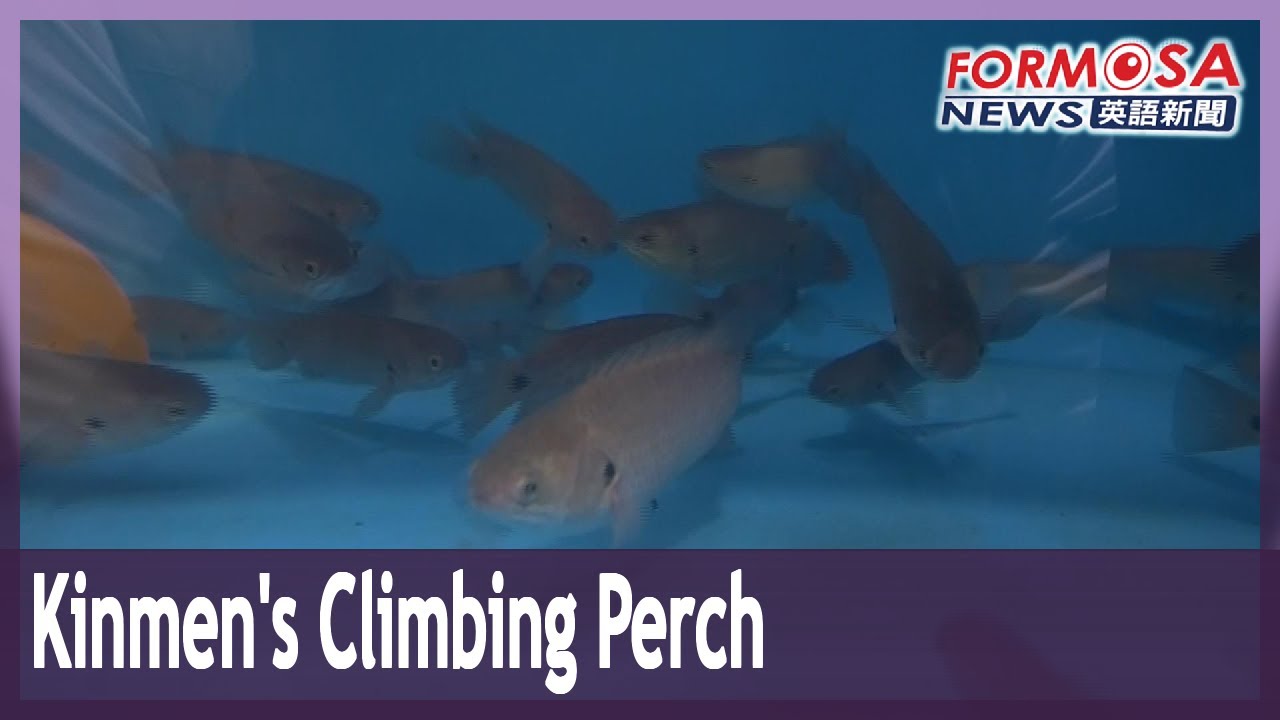The image features a rectangular layout with a wider perspective, emphasizing its horizontal dimension. The borders are framed by a thin purple outline on the top, left, and right sides, while the bottom section features a thicker dark purple border. This bottom border contains white text that reads "Kinmen's Climbing Perch." In the upper right corner, "Formosa" is prominently displayed in red text, followed by "News" in black text with some accompanying Asian characters.

The central image captures a medium-sized fish tank or aquarium, as indicated by the reflections on the glass. The tank's water has a medium to dark blue hue, and the bottom is light blue and clean. Inside, around 15 small to medium-sized fish, identified as perch, swim in various directions. These fish are generally gray or tannish-brown in color, contributing to the tranquil underwater scene.